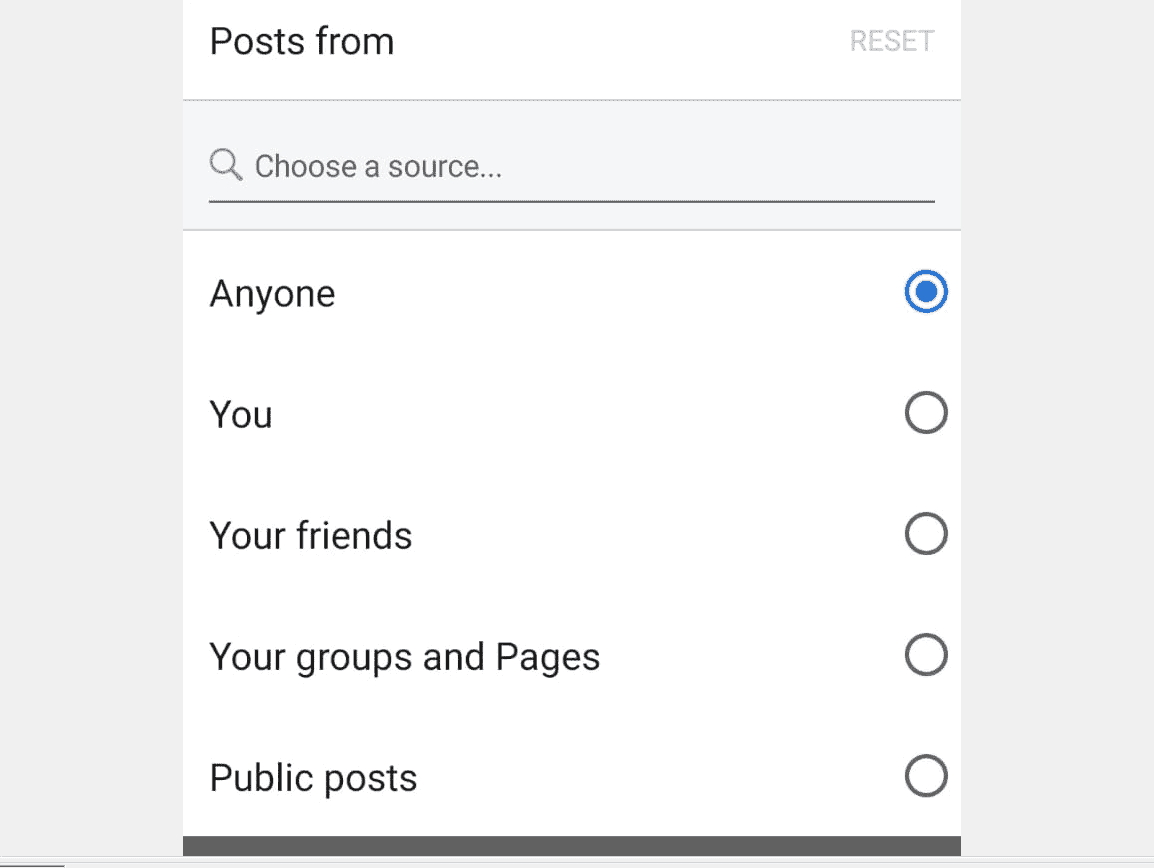The screenshot features a user interface with a gray background. Prominently displayed are two buttons: 'Post', which is highlighted in black, and 'Reset', which is shaded in gray. Toward the upper corner, there is a magnifying glass icon, indicating a search function. Below this, the option to 'Choose a source' is visible, accompanied by a series of radio buttons aligned to the right.

Among these options, 'Anyone' is selected and highlighted in blue, signifying it as the current choice. Additional options include 'You,' 'Your Friends,' 'Your Groups and Pages,' and 'Public Posts,' listed beneath 'Anyone.' These options are associated with corresponding radio buttons, which are not currently selected.

At the bottom of the interface, there is a black rectangle that appears to function as a footer or perhaps an action button section. This is immediately followed by a gray scroll bar located at the very bottom of the screenshot, indicating more content available beyond the visible area.